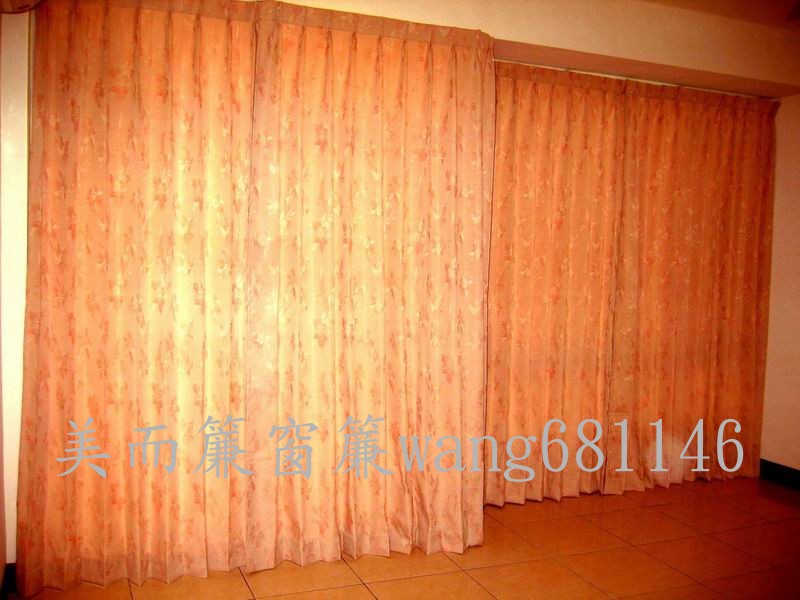The image depicts an interior room featuring dominant shades of orange. Central to the composition is a sanded orange column with matching walls on either side. The floor consists of large orange tiles, transitioning from a yellow tint on the left to a more pronounced orange hue on the right. On the far wall, elegant light-to-dark orange curtains, adorned with a ridge-like pattern and topped with folded fabric, extend to the floor. The curtains on the left project further into the room compared to those on the right, possibly indicating a glass panel or a sliding mechanism behind them. Along the cream-colored walls with a dark baseboard, there's noticeable grey writing in both an Asian script and English, reading "WANG 681146." These characters, partially obscured, suggest a watermark, running about 80% of the way down the left side of the image. Sunlight appears to filter through the curtains, casting a shimmering, golden glow across the scene.